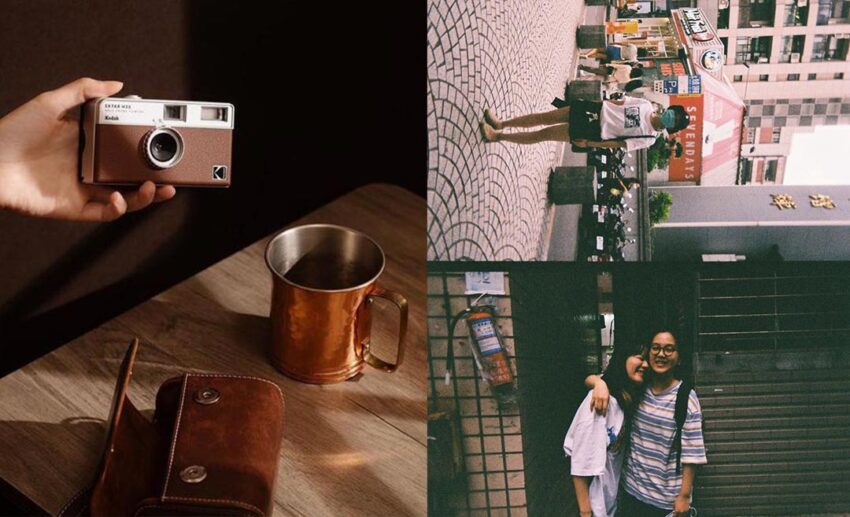The image is a detailed collage consisting of three panels. The left panel, which occupies the entire left side, features a close-up of a person's hand holding a vintage Kodak film camera above a wooden table. On the table, there's a copper mug, along with a leather case presumed to belong to the camera. The top right panel displays a woman standing in a plaza with pavers below. She wears shorts, a white t-shirt, a COVID mask, and a cap, with a handbag over her left shoulder. The scene includes both small tented structures and larger buildings in the background. The bottom right panel depicts two women arm-in-arm, smiling and hugging. One woman wears circular glasses and a blue striped shirt, while the other wears a long white t-shirt. They appear to be in front of a shop, with visible details such as a fire extinguisher and a metal grate. All images are in bright natural lighting, enhancing their clarity. The collage intricately merges these moments into a cohesive narrative.